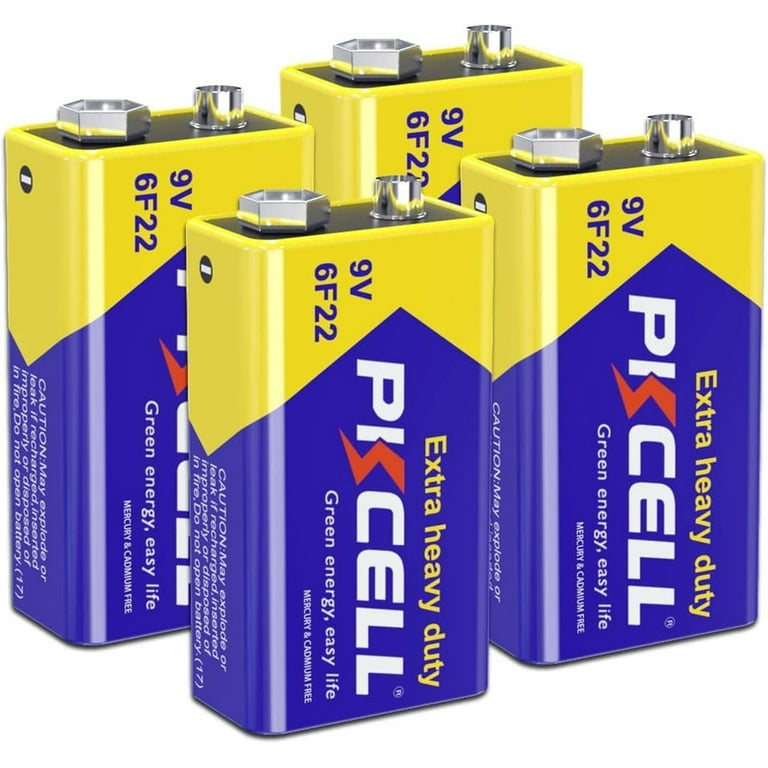This is a close-up image of four identical 9-volt PISCELL batteries against a featureless white background, arranged in a 2x2 formation with two standing in the front and two behind them. Each battery is a vertical rectangle, narrower from front to back than they are across. The top portion of the batteries is yellow, where the positive and negative connections are located, bordered by an upside-down V-shaped or sawtooth pattern. The majority of the battery's body is blue and features the branding and descriptive text. Displayed parallel to the long side in white font, the brand name "PISCELL" is split by a red lightning bolt. Below the brand name, in smaller yellow and white fonts, are the words "extra heavy duty" and the tagline "green energy, easy life." Some batteries also have additional small text indicating they are mercury and cadmium free, and display "9-volt 6F22." All the batteries are aligned in the same direction, although some appear to be slightly taller than others, potentially revealing part of a caution warning on their sides.